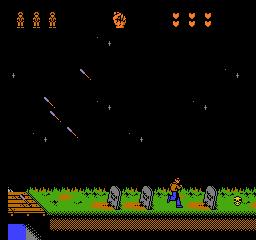In the video game screenshot, a humanoid character is depicted running through a somber graveyard. The ground is covered in grass, interspersed with gravestones carved from gray stone, each gravestone protruding from the grassy surface with a patch of orange dirt in front, creating an eerie ambiance. The gravestones are etched with black markings, mimicking writing but devoid of real text. The figure, wearing an orange long-sleeve shirt, blue jeans, and matching blue shoes, moves from left to right between two of the gravestones. In total, three gravestones are visible amidst the scene. Behind this grassy graveyard lies a brown wooden bridge. The night sky forms the backdrop, painted in black and dotted with white stars, some of which form small crosses, and streaks of light representing shooting stars or space debris. At the top of the screen, orange icons display crucial player information, adding to the immersive gaming experience.